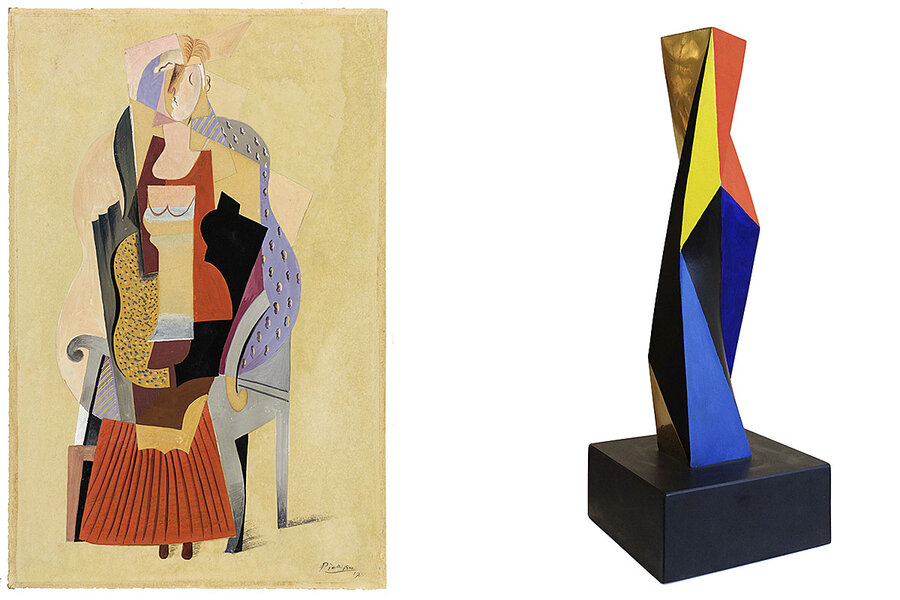The image showcases two pieces of abstract art side by side. On the left, there is a drawing resembling the work of Picasso, evident from the signature in the bottom right-hand corner. This artwork is rendered on yellow-hued paper and vividly portrays a woman seated in a blue chair, dressed in a long, brick-red dress. The woman has her eyes closed, and intricate shapes and details such as a fan on her right side are interwoven within the composition. The drawing features a mix of colors including reds, yellows, blues, grays, and blacks, capturing Picasso's renowned use of geometric forms and abstract elements.

To the right of the drawing is a sculpture presented on a black square base. This abstract sculpture is geometric and twisted in form, composed of various colors like orange, yellow, blue, light blue, black, and brown. The sculpture lacks a visible signature or any identifying mark, adding an element of mystery to its origin. Both pieces of art, placed side by side, offer a vibrant and multifaceted exploration of abstract expression through different mediums.